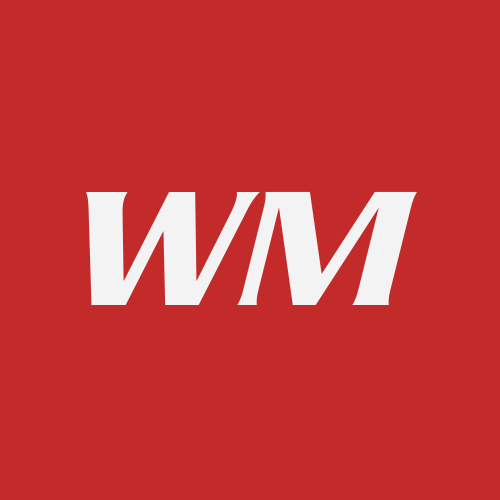The image showcases a striking logo set against a solid primary red background, which fills the entire frame without any shadows or gradients. In the center are the large white block letters "W" and "M," displayed in an italicized, capitalized font. These letters are designed to mirror each other vertically, creating a symmetrical appearance if the logo were flipped top to bottom. The "W" and "M" feature hard, angular lines with subtle serifs at the ends. Notably, the left side of the "M" is narrower than its right side, with the left middle section being thicker than the right middle. The letters lean slightly from the lower left to the upper right, adding a dynamic feel to the simple yet bold design.